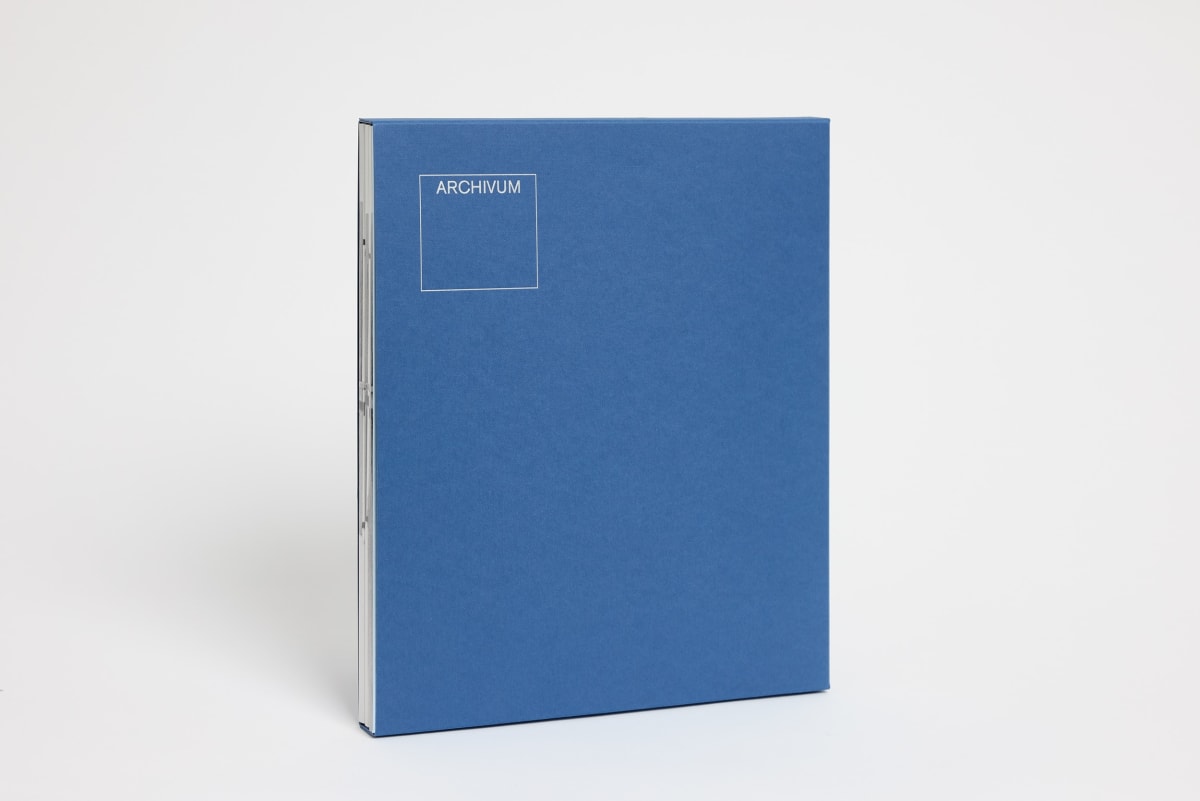This image features a sleek, medium-blue binder or notebook standing upright against a pure white background. The notebook, approximately half an inch thick, is angled slightly to the side, revealing white pages or possible album-style sleeves inside. The front cover prominently displays a white square in the top left-hand corner with the brand name ARCHIVUM in bold, uppercase letters. The minimalist background and clean design underscore the promotional nature of the photo, emphasizing the binder's elegant and functional appearance.